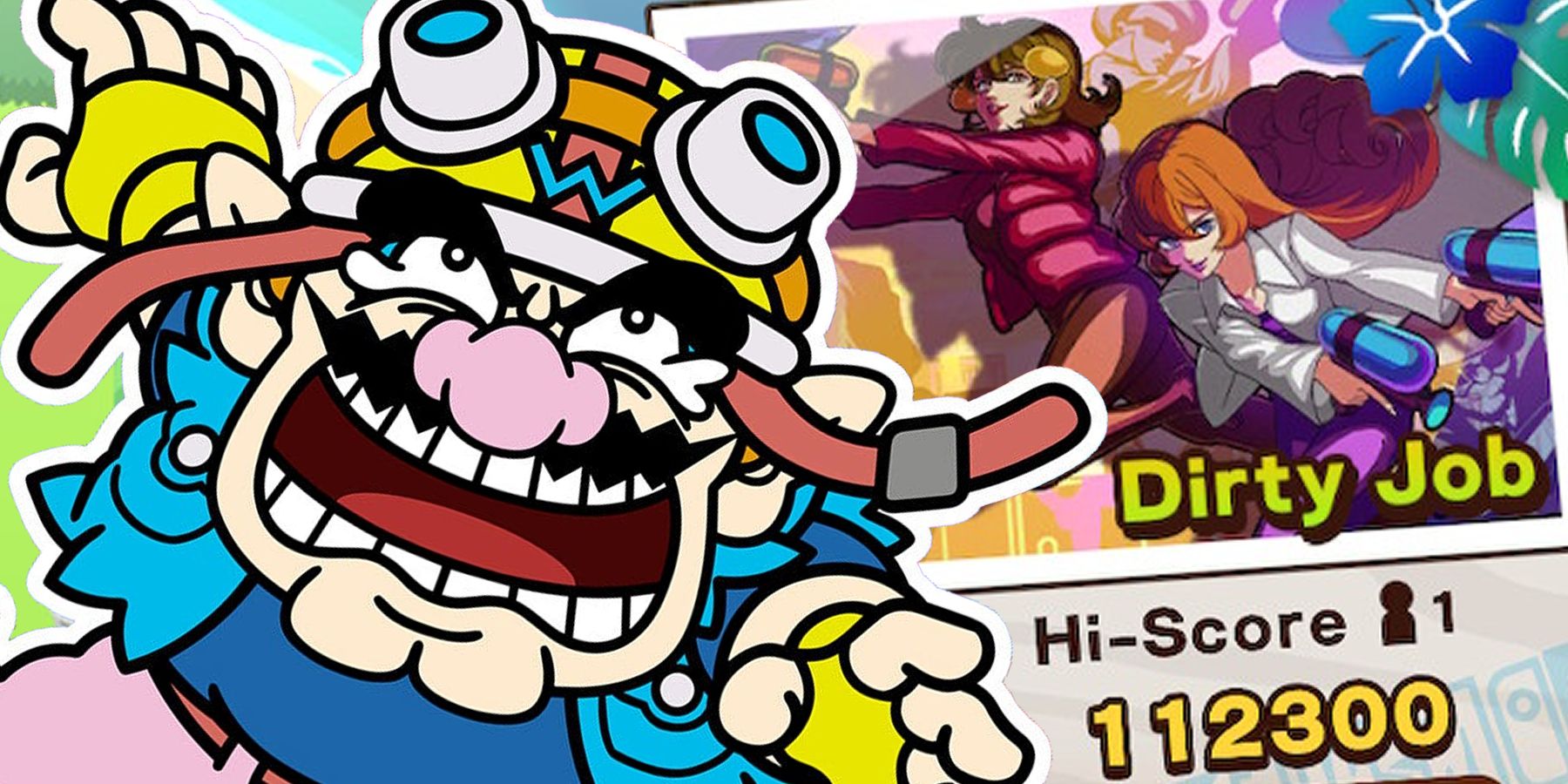The image depicts a vibrant, colorful video game screen featuring a mix of characters from different visual styles. On the left side, a large, exaggerated figure resembling Wario from the Mario Brothers franchise is depicted. Wario is adorned in a pilot's cap with yellow, red, and orange hues, featuring a prominent blue "W". His attire includes yellow fingerless gloves, a blue vest, and matching blue pants, while his facial details boast thick, black lightning-bolt eyebrows, a distinctive black mustache, and an open mouth showcasing his teeth and tongue. Wario's comically large chin, pink cartoonish nose, and elf-like ears add to his exaggerated look.

On the right side of the screen, two anime-style women are illustrated in a different artistic style. They are each holding water guns and have pronounced features such as detailed hair, waists, hips, and arms. Surrounding them are vibrant tropical flowers that enhance the lively and colorful theme of the image. The bottom right corner of the screen displays the text "Dirty Job" followed by "High Score" and the impressive score of either 1,123,000 or 112,300, with a small icon of a person marked as number one beside the score. This screen amalgamates bright and dynamic elements from both video game and anime genres, creating an eye-catching and playful scene.